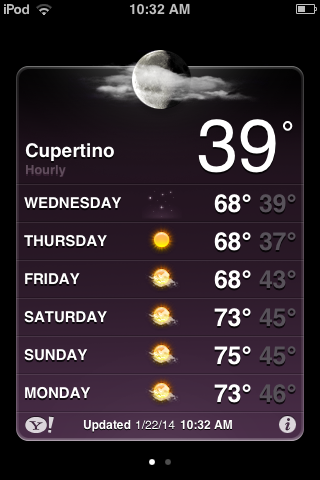This is a detailed caption for the described image:

---

The image is a screenshot depicting a weather forecast on a black background. At the top of the screen, in white text, "iPod" is displayed with the 'i' in lowercase, followed by 'P' in uppercase and 'od' in lowercase. The top bar also shows the Wi-Fi signal strength on the left, the current time, "10:32 AM," in the center, and the battery icon, which is half-filled, on the right.

Beneath this, a thin-lined, rounded-edged square contains an image of the moon. The moon appears with its dark side on the right and its bright, illuminated part on the left, partially covered by clouds.

Below the image, the weather details in white text read: "Cupertino, 39°," followed by the label "Hourly."

Further down, detailed daily forecasts are provided:

- **Wednesday:** Sunny, 68° high, 39° low.
- **Thursday:** Sunny, 68° high, 37° low.
- **Friday:** Partly cloudy, 68° high, 43° low.
- **Saturday:** Partly cloudy, 73° high, 45° low.
- **Sunday:** Partly cloudy, 75° high, 45° low.
- **Monday:** Partly cloudy, 73° high, 46° low.

At the bottom of the image, the Yahoo Weather symbol is visible, consisting of a circle with a 'Y' and an exclamation point. The forecast appears to be updated as of "1-22-14, 10:32 AM."

---